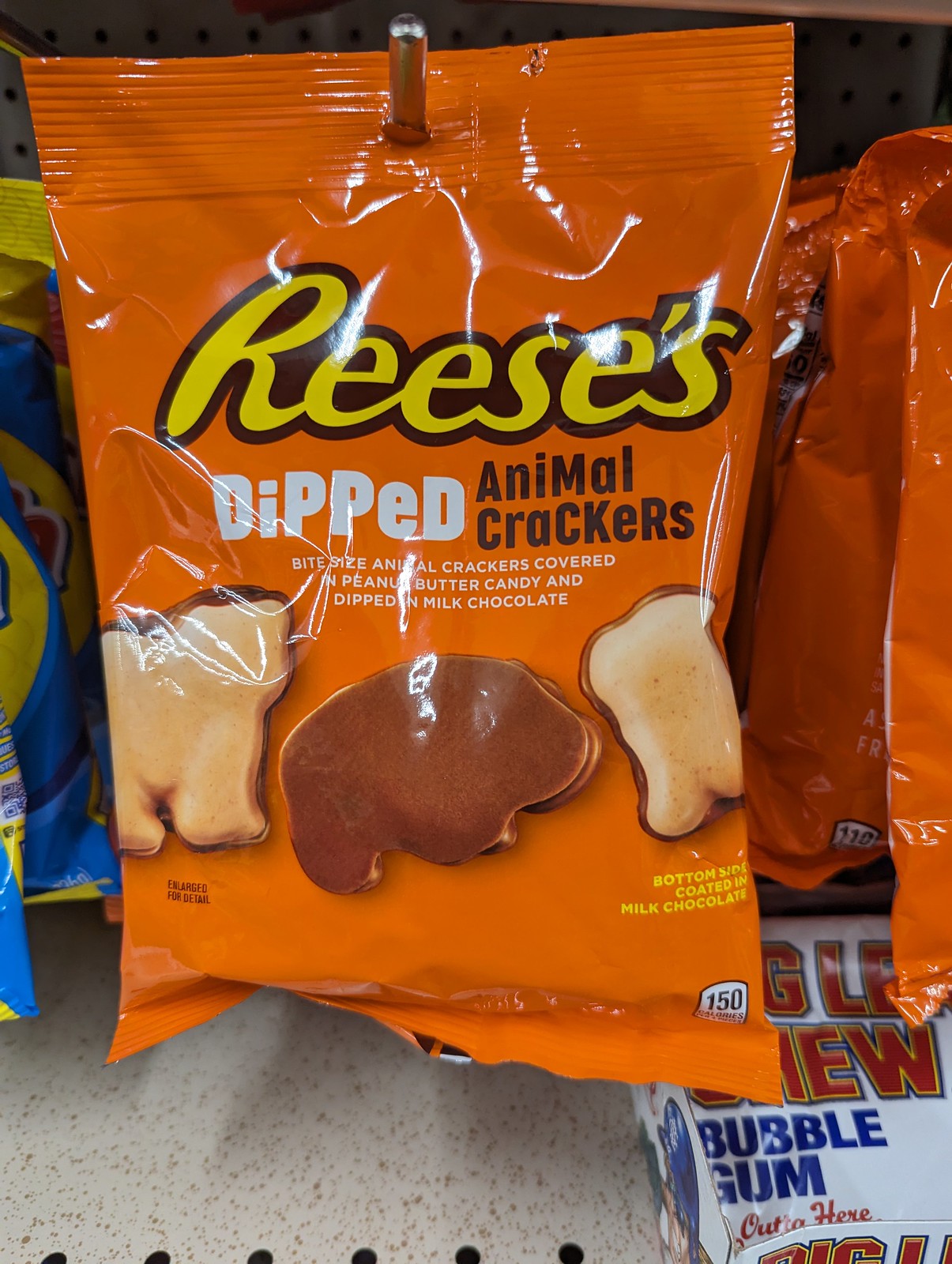A meticulously organized store display features an eye-catching orange bag of Reese's Dipped Animal Crackers prominently hanging on a rack. The vibrant packaging, emblazoned with the iconic Reese's logo, showcases appetizing images of animal crackers covered with chocolate on top and filled with luscious peanut butter in the middle. Surrounding the Reese's bag are similar confectionery items, each neatly aligned on either side. To the bottom right of the display, a box of Big League Chew Bubble Gum is visibly perched on a shelf, adding to the array of sweet treats. The scene captures the inviting ambiance of the candy aisle, with an array of brightly colored packages that entice shoppers with their delectable offerings.